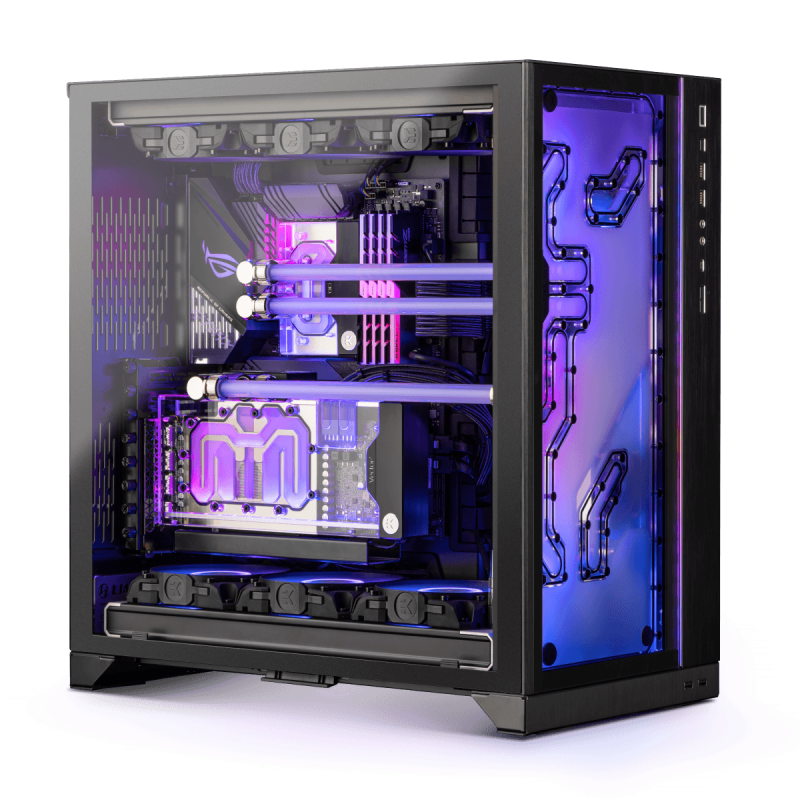This image showcases a highly detailed and custom-built desktop PC within an all-black, tempered glass case that beautifully displays its internal components. The standout feature is the ASUS ROG motherboard, illuminated by purplish-pinkish RGB lighting, which matches the neon coolant flowing through the custom loop cooling system. This intricate system includes a custom radiator at the front, with three tubes leading from the radiator to the CPU and GPU, each cooled separately. Additionally, the system boasts four sticks of RAM, also illuminated in purple RGB, and complemented by the six RGB fans—three at the bottom and three at the top of the case. 

The ASUS ROG logo on the motherboard shines in a matching purple hue, echoing the RGB aesthetics. Custom purple cable sleeves add an extra layer of sophistication. The tower’s exterior is adorned with a vibrant, patterned purple design, evoking the intricate appearance of a silicon chip, highlighted by clear lines that cross the surface. 

On the top right corner of the case, multiple USB and auxiliary ports are visible, as are additional USB ports on the bottom right. The clear tempered glass side panel allows an unobstructed view of these meticulously arranged internals, showcasing the powerful components and the elegant, cohesive color scheme of the custom build.